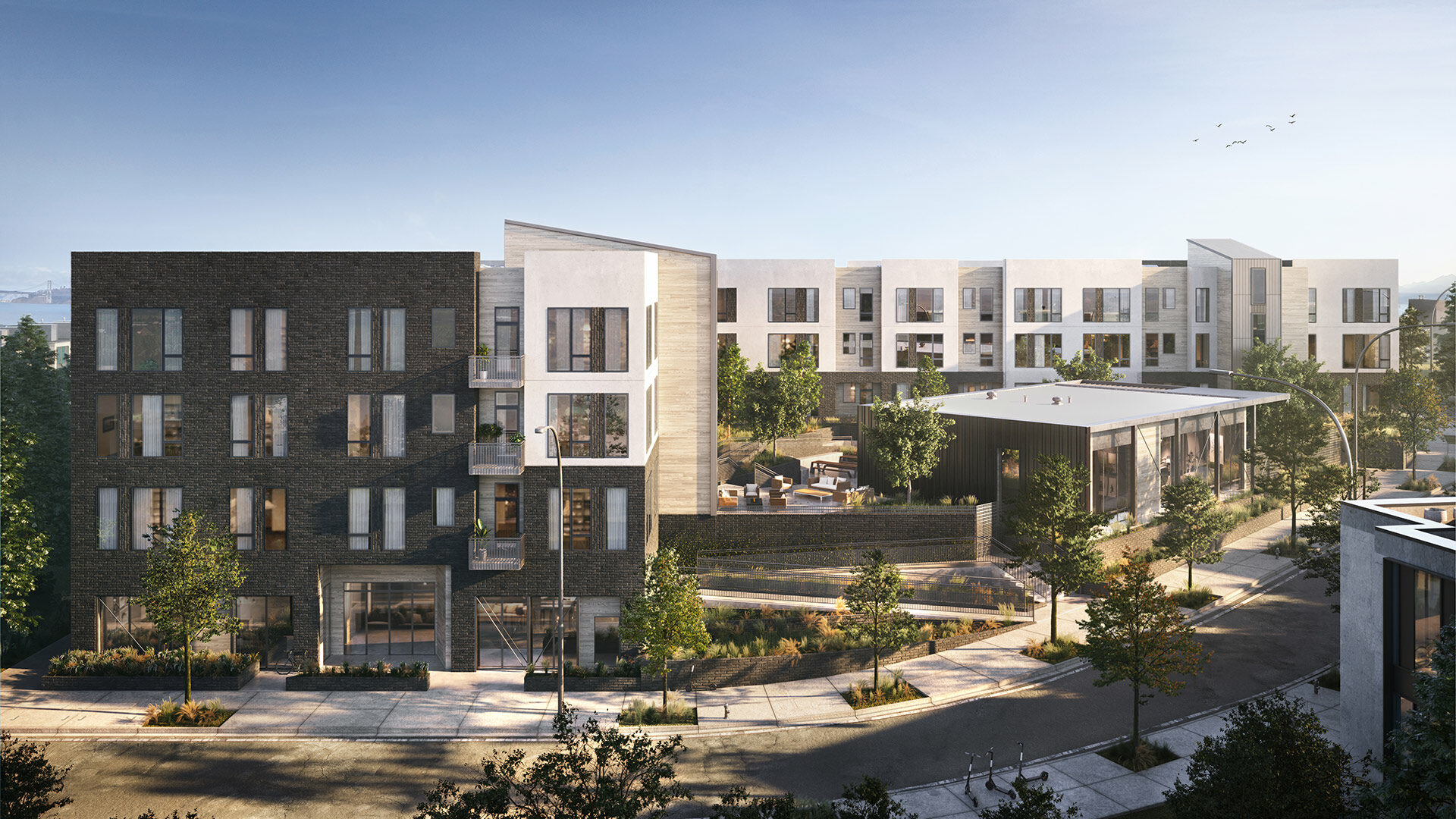The image depicts a surreal, potentially computer-generated or model-like, street scene showcasing a modern residential area. The setting features numerous upscale apartment complexes characterized by a mix of dark gray and white bricks. The buildings, which appear to be new and contemporary, rise up to four stories, some with balconies and others without. The photograph is taken from an elevated viewpoint, offering a wide, panned-out view of the area, which includes neatly designed sidewalks made of white cement, arranged in broad, inviting pathways.

Notably, the scene is devoid of any cars, bicycles, or people, which enhances the surreal quality of the image. The street curves gently around the complex, and young, thin trees, almost like saplings, are planted in rectangular beds along the sidewalks. These trees have green leaves, adding a touch of nature to the urban landscape. To the left, a main building stands prominently, while more apartment complexes stretch into the background on the right, with a smaller structure that could be a clubhouse nestled amid communal space featuring wicker-style furniture.

The area appears meticulously planned, possibly for use by architects or city planners, and includes streetlights spaced along the road. The sky above is a gradient of light blue to a slightly darker hue, accentuating the clean and modern atmosphere of this envisioned or model-designed community.